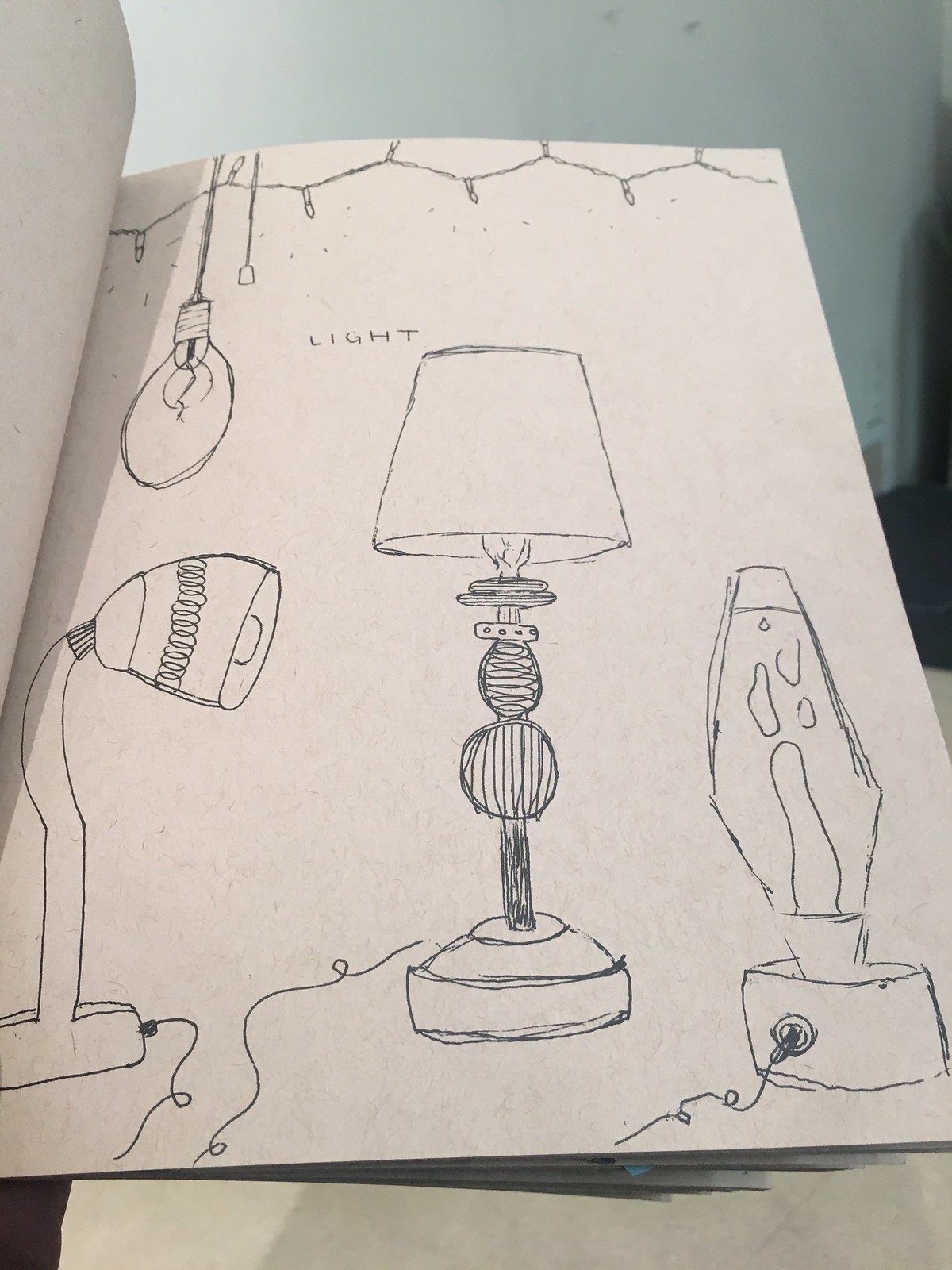In this portrait-oriented photograph, a white sketchbook is open, revealing a detailed black and white pencil sketch on the right-hand page. The left-hand page is slightly folded, casting a subtle shadow over the illustrated page, adding depth to the composition. Central to the sketch is an intricate drawing of an elegant lamp with a circular base and a narrow pole that transitions into a spherical element, topped by another sphere and crowned with a traditional lampshade. In the upper left corner, an overhanging light bulb is meticulously sketched, lending a sense of functional ambiance to the scene. To the left, a small table lamp is depicted, balancing the composition, while the right corner features a curvaceous lava lamp, adding a playful contrast. Each lamp is drawn with accompanying extension cords, although their destinations are artistically left to the viewer’s imagination. Above the assortment of lamps, a string of Christmas light decorations is delicately penciled, evoking a sense of festivity and warmth. The overall composition is both charming and detailed, capturing a whimsical yet cozy tableau of various lighting elements.